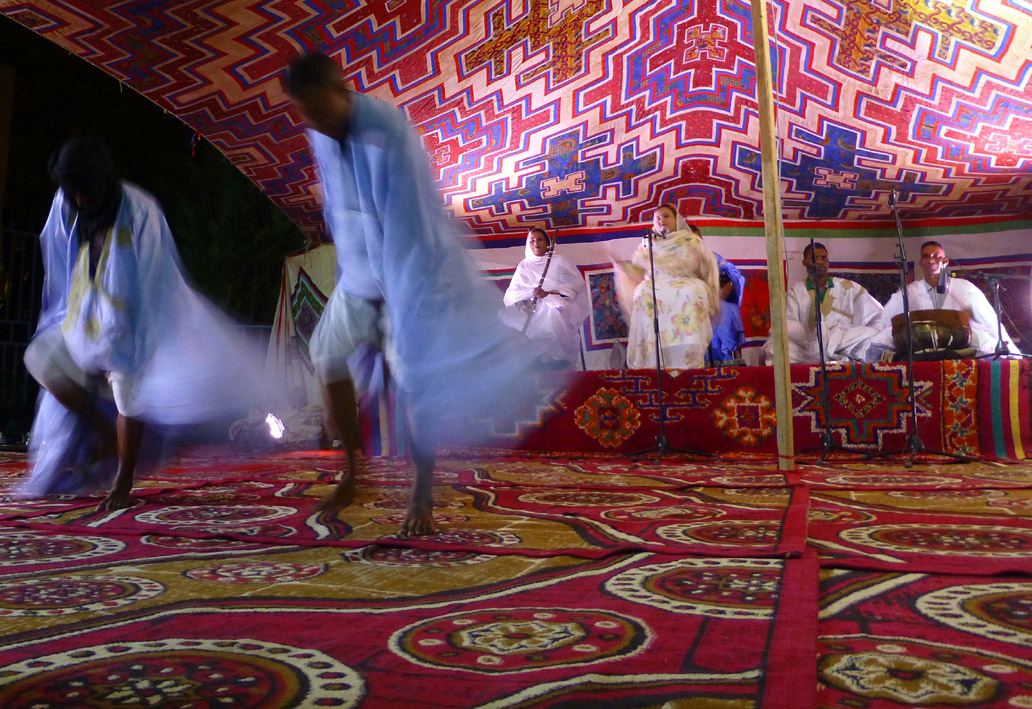This vibrant photograph captures the lively scene inside a tent, possibly set in India or the Middle East, illuminated by an array of colorful patterns and designs. The tent's ceiling is adorned with bright, abstract geometric shapes, primarily in red and blue, held up by a central pole. The floor is covered with multicolored rugs featuring intricate, geometric patterns in red, dark yellow, and white.

At the heart of the scene, a lady dressed in an ethnic outfit stands on a stage, passionately singing into a microphone. Beside her, another woman, also attired in traditional clothing, plays a wind instrument, possibly a reed-like instrument. Flanking them are two men with dark hair; one plays a drum, contributing to the rhythmic heartbeat of the performance, while the other stands without any visible instrument. Another individual can be seen behind the lady singing, adding depth to the ensemble.

In the foreground, two dancing figures, dressed in flowing blue robes, move energetically across the floor. Although they appear blurry due to their dynamic motion, their bare feet and rhythmic movements add to the festive atmosphere. The backdrop features pictures on the wall, enhancing the cultural richness of the setting. Overall, this image encapsulates a vivid and colorful celebration filled with music, dance, and traditional attire, suggesting a possible wedding or a cultural event taking place at night.